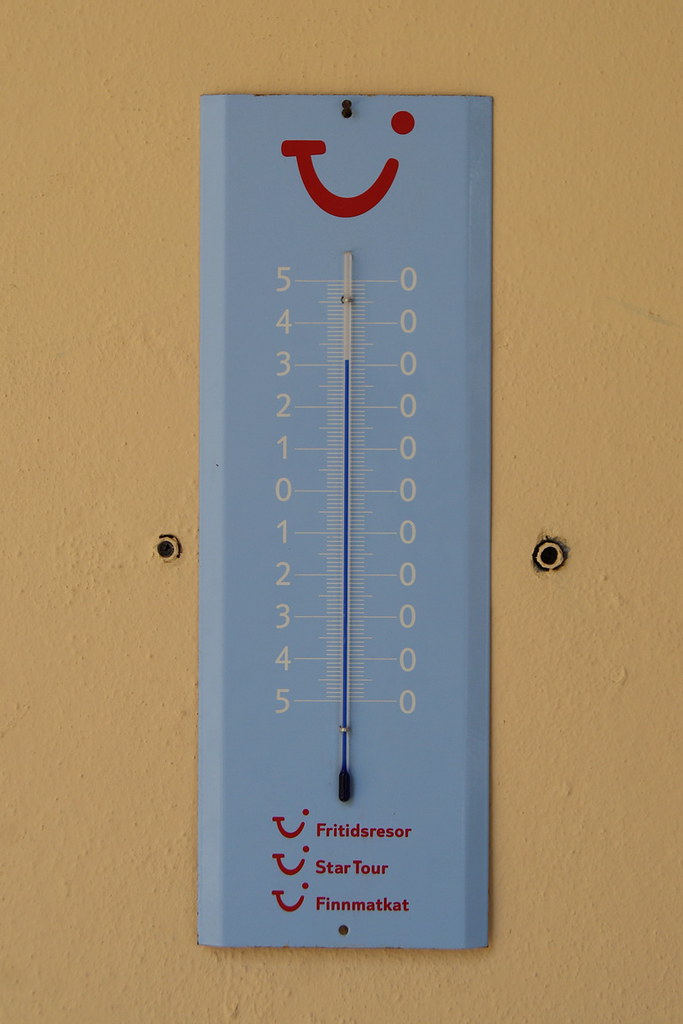A light brown, foot-long piece of wood serves as the base for a vivid blue thermometer. Each end of the wood features a slightly rusty hole, adding a touch of character. The thermometer, positioned centrally on the log, boasts a red smiley face at the top, complete with two small red eyes and a cheerful smile. The thermometer itself is encased in a white and clear body, with temperature markings running along both sides. The right side displays a series of zeros, while the left side is marked with numbers from 5 down to 0 and back up to 5 in white. At the bottom of the thermometer are three red semi-smiley faces, each accompanied by a different label: "Fritigrass," "Star Tour" with a smiley face, and "Finn Matkett" with another smiley face.